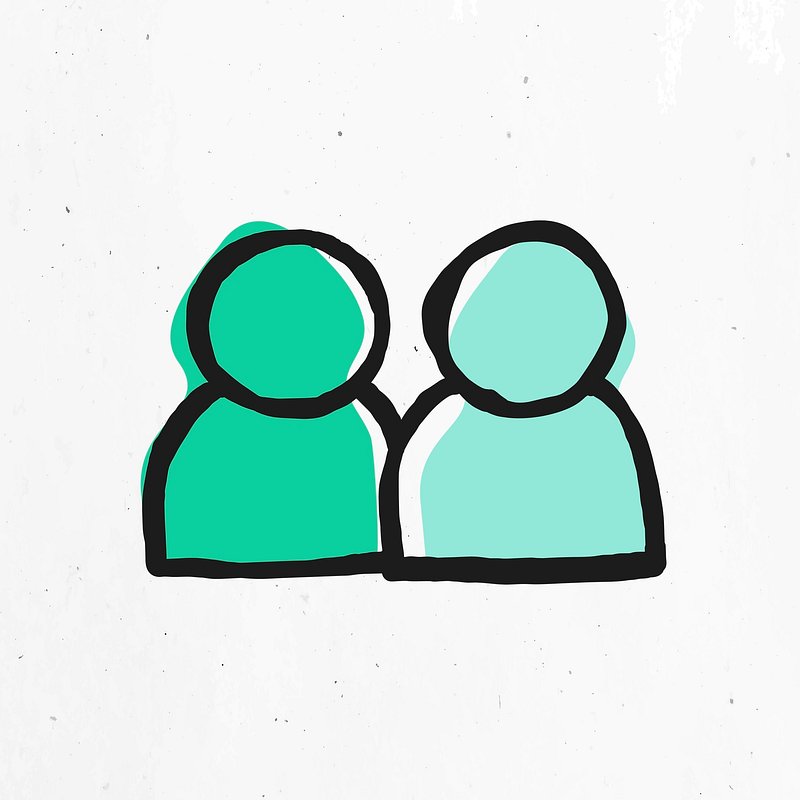The image resembles a children's drawing or a stylized digital illustration, featuring two simplistic human figures on a white background scattered with tiny black specks. Each figure consists of a black circle for a head and a half-circle or pill-shaped torso. The left figure has a black head and torso, filled unevenly with a green color that spills out, leaving some white areas within the shapes. Behind and around this figure is a green background. The right figure mirrors the left but is filled with a lighter green or teal shade, also spilling beyond its borders and leaving some white spots. Both figures convey a sense of simplicity and messiness in their uniform yet flawed application of color.